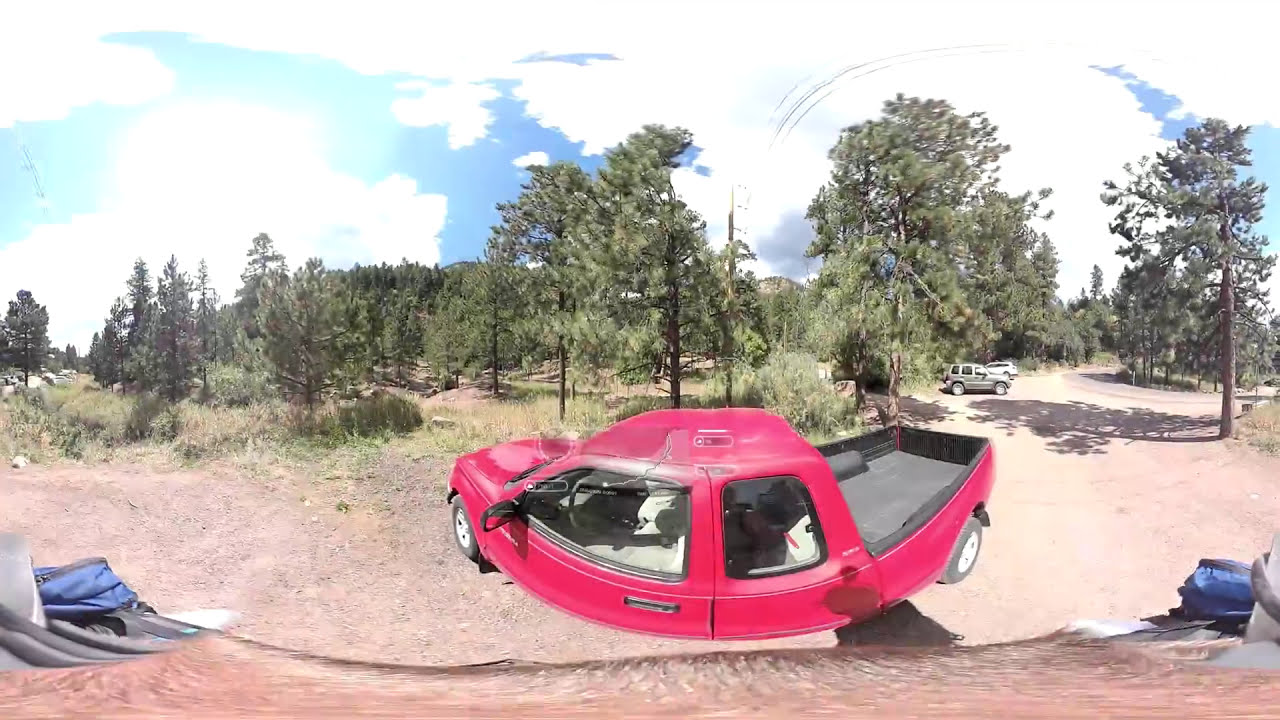This panoramic outdoor scene captures a 360-degree view, revealing a wide stretch of landscape and sky. At the center of the image is a heavily distorted and curved bright red extended cab pickup truck with a black bed liner, parked on a dirt and gravelly area. This distortion gives the truck an almost smiley face appearance. The foreground features a brown, unidentifiable object stretched across the bottom of the picture.

In the background, under a light to dark blue sky dotted with bright white, somewhat glary clouds, stands a mix of tall trees, including evergreens and some with green leaves. To the left of the truck, the area is filled with grass and more trees. On the right, extending into the distance, there is a dirt road or parking area where several other vehicles, including a silver car and a white SUV, are parked. This road or parking area, lined with tall trees on either side, adds depth to the expansive scene.